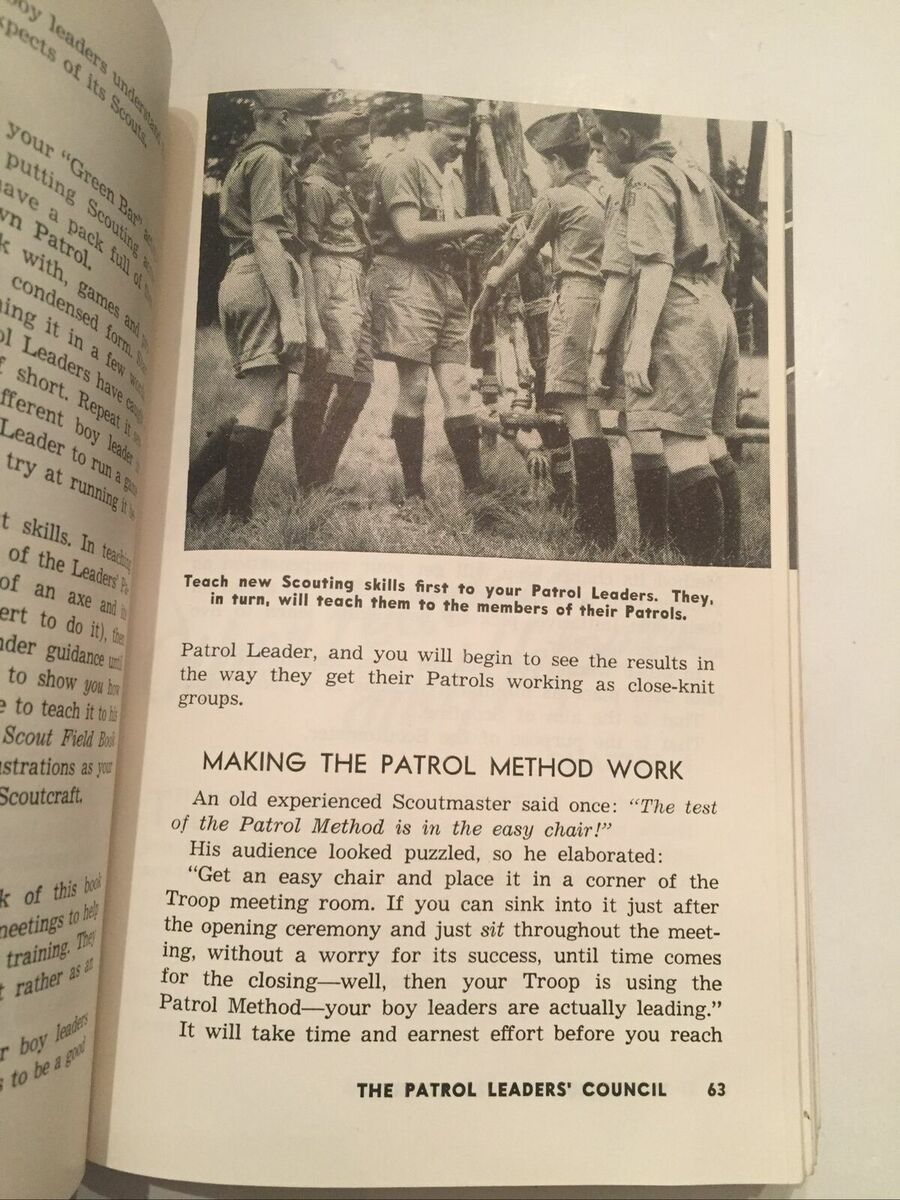The photograph depicts a yellowed, worn page from a vintage Patrol Leaders Council handbook, likely from the Boy Scouts, captured lying open on a cream-colored surface. The page, numbered 63, showcases a black-and-white image of scouts outdoors, dressed in traditional uniforms consisting of knee socks, long shorts, short-sleeve shirts tucked in, hats, and the iconic scouting handkerchiefs tied around their necks. The scouts, including one adult leader, appear to be engaged in a project. The caption beneath the image reads: "Teach new scouting skills first to your patrol leaders. They, in turn, will teach them to the members of their patrol." Additionally, the page includes text emphasizing the patrol method's effectiveness, highlighted by the anecdote of a wise scoutmaster who states that a successful troop allows a leader to sit back and relax in an easy chair, assured that the boy leaders are independently guiding their patrols. The heading "The Patrol Leaders Council" is prominently displayed on the bottom right of the page.